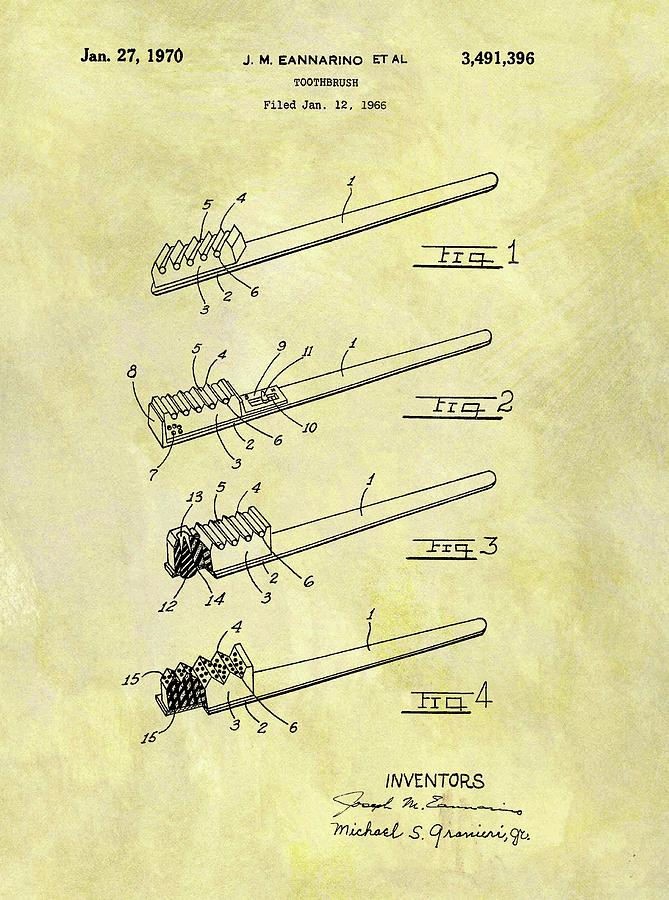The image depicts a detailed diagram for a patent application of a toothbrush, filed on January 12, 1966, and reprinted on January 27, 1970. The top left corner features the date "January 27, 1970," and the middle top section includes the name "J.M. Annarino et al." This document, labeled with the patent number 3,491,396, outlines various views of the toothbrush across four figures, each marked with "Fig. 1," "Fig. 2," "Fig. 3," and "Fig. 4." The depictions reveal a toothbrush handle with a solid material on top, differing from traditional bristles. Each figure is annotated with numbered callouts identifying different components. At the bottom, the inventors' signatures, Joseph M. [illegible], and Michael S., are visible, emphasizing the collaborative effort. The paper is aged, hinting at its historical significance in toothbrush design evolution.